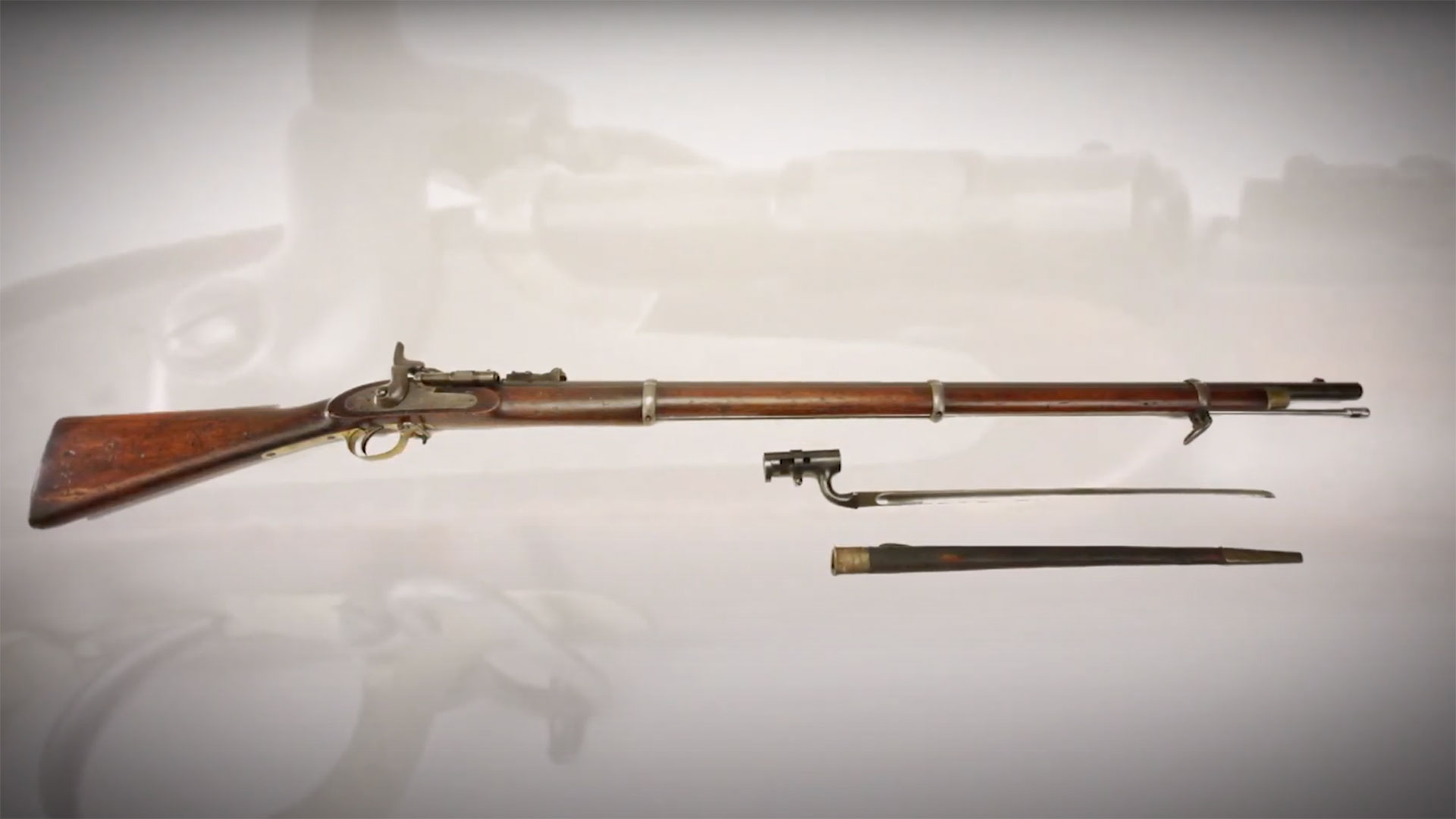This image features an old-fashioned rifle with a wood exterior, showcasing a classic, long-barreled design reminiscent of an old Western-style shotgun or musket. The rifle, centered prominently in the frame, is made of brown wood and has an elaborate metal mechanism near its butt, including the trigger and the chamber-loading component. Accompanying the rifle are several accessories: beneath it lies a nickel-colored gun cleaning tool with a straight, coat-hanger-like design, and just below this tool, there’s a brown cover that possibly has a copper tip. Additionally, there appears to be a sword-like device, adding to the assortment of tools. The backdrop features a faded, close-up image of the trigger area, blending subtly into the light white and gray-toned background, with gray shading accentuating the four corners of the picture.